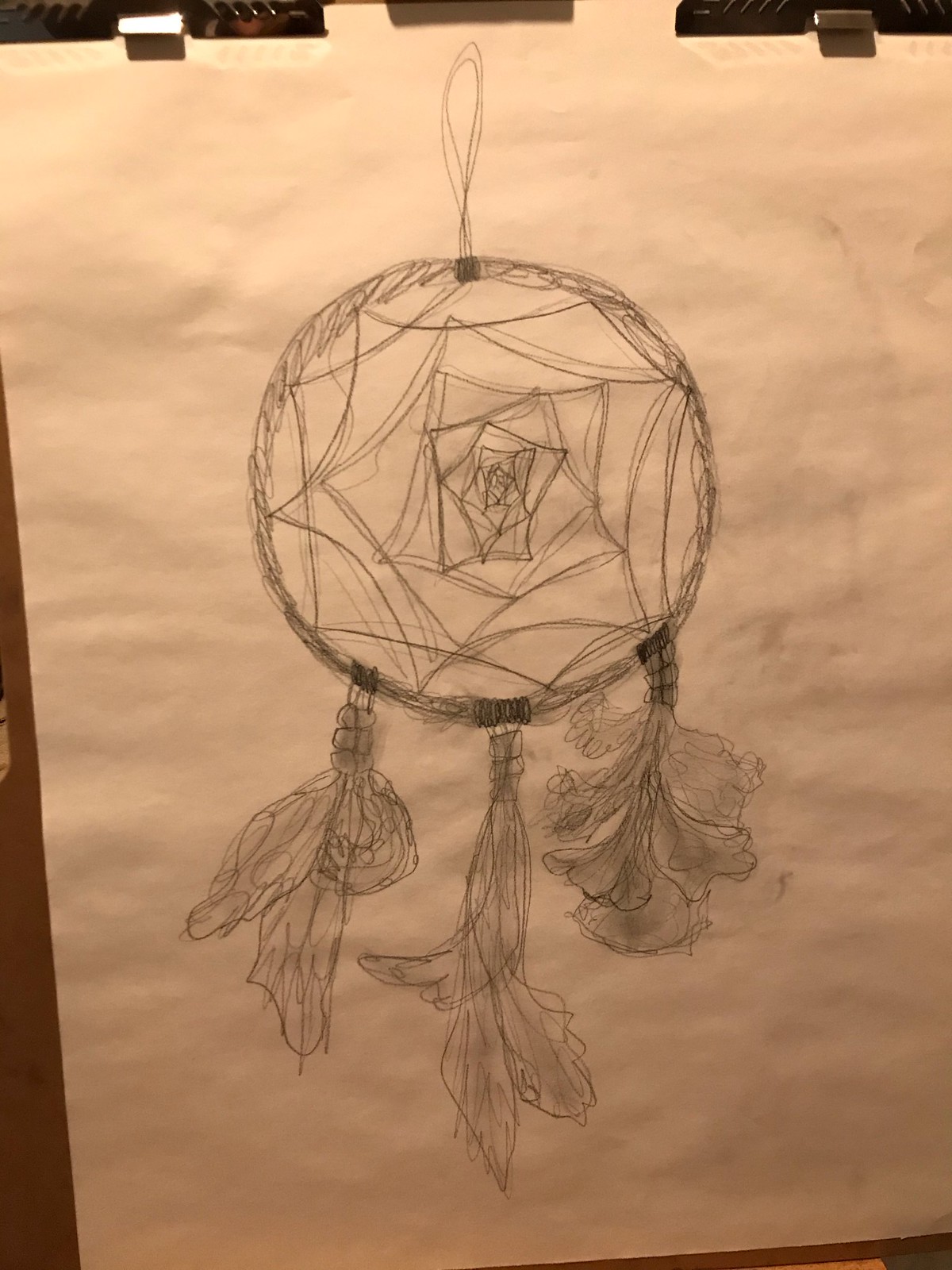A meticulously detailed pencil drawing of a dreamcatcher is presented on a pristine white sheet of paper, securely fastened at the top with two clips. The dreamcatcher features a hoop at its apex, suggesting it is designed to be hung. The primary section of the dreamcatcher is a circular web, intricately woven with curving lines resembling a spider's web. Emerging from the bottom of the circle are three elaborate extensions, each adorned with intricate feather-like designs brimming with squiggly line patterns. These extensions vary slightly in detail, with the one on the far right boasting five or six feathers, compared to the other two sections which each have three feather-like elements. The drawing showcases areas of darker shading, notably appearing like coils, adding depth and dimension to this beautifully rendered piece.